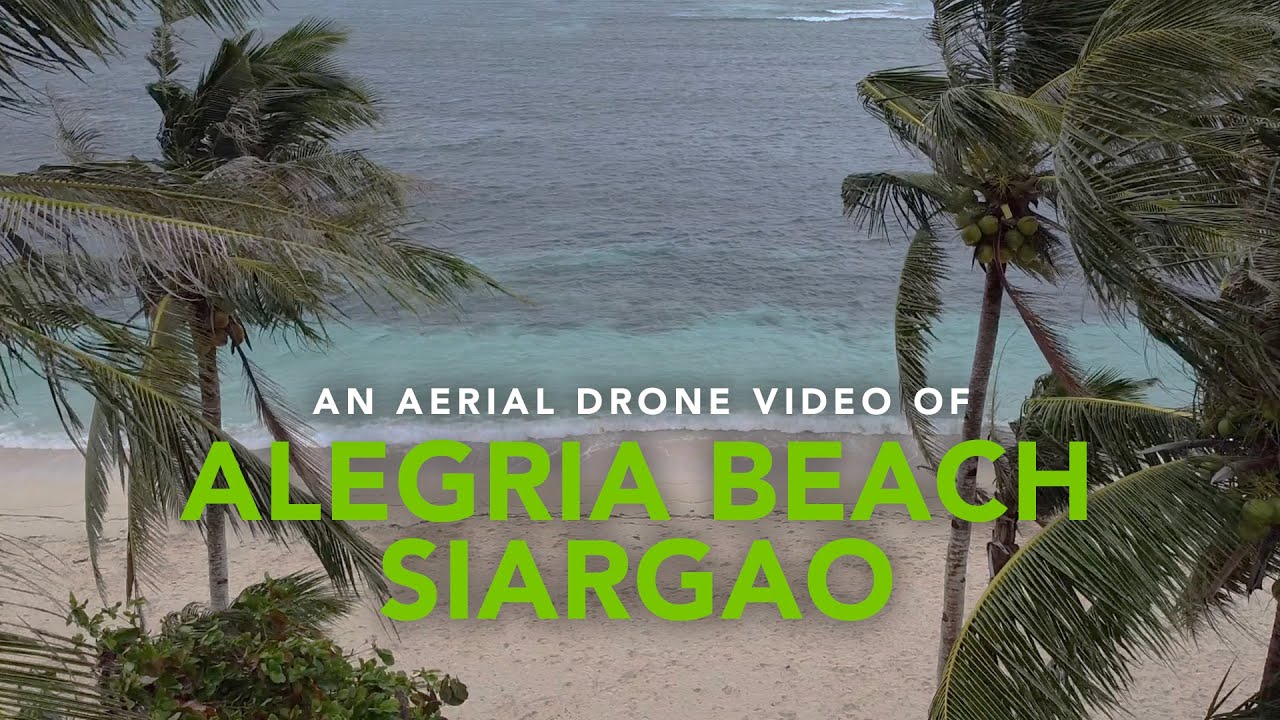The image captures an aerial view of Alegria Beach, Siargao, likely serving as a thumbnail for an upcoming video. This serene and picturesque beach, devoid of people, seems to have been photographed early in the morning. The water near the shore appears as a clear, light turquoise that deepens to darker shades further out, indicating potential coral or rocks below. The sandy beach is pristine, free from debris, and offers a welcoming sight for potential tourists. Flanking the beach on either side are clusters of palm trees and coconut trees, their fronds swaying vigorously in the wind. The center of the image is dominated by text: "An aerial drone video of" in bold white letters, followed by "Alegria Beach" in large, bold lime green text, and underneath that, "Siargao" in white. The lush greenery, combined with the inviting waters, make this coastal spot a promising destination for beachgoers.